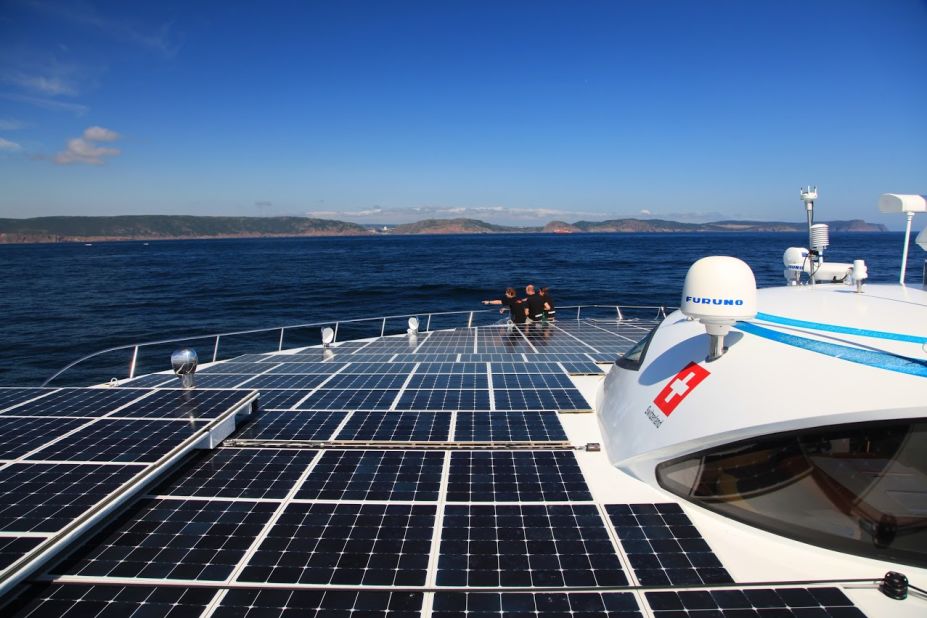The image showcases a large solar-powered boat with a top deck covered in blue solar panels featuring white lines. At the bow of the boat, three people dressed in black outfits sit with their feet hanging over the edge, pointing towards the calm, dark blue sea. They lean against a silver safety bar. Towards the right side of the boat, there is a white section with a red square featuring a white cross, labeled "Switzerland" underneath. A window is also present on this white part. In the background, brown and green mountains rise from the water's edge, adding to the serene marine setting.